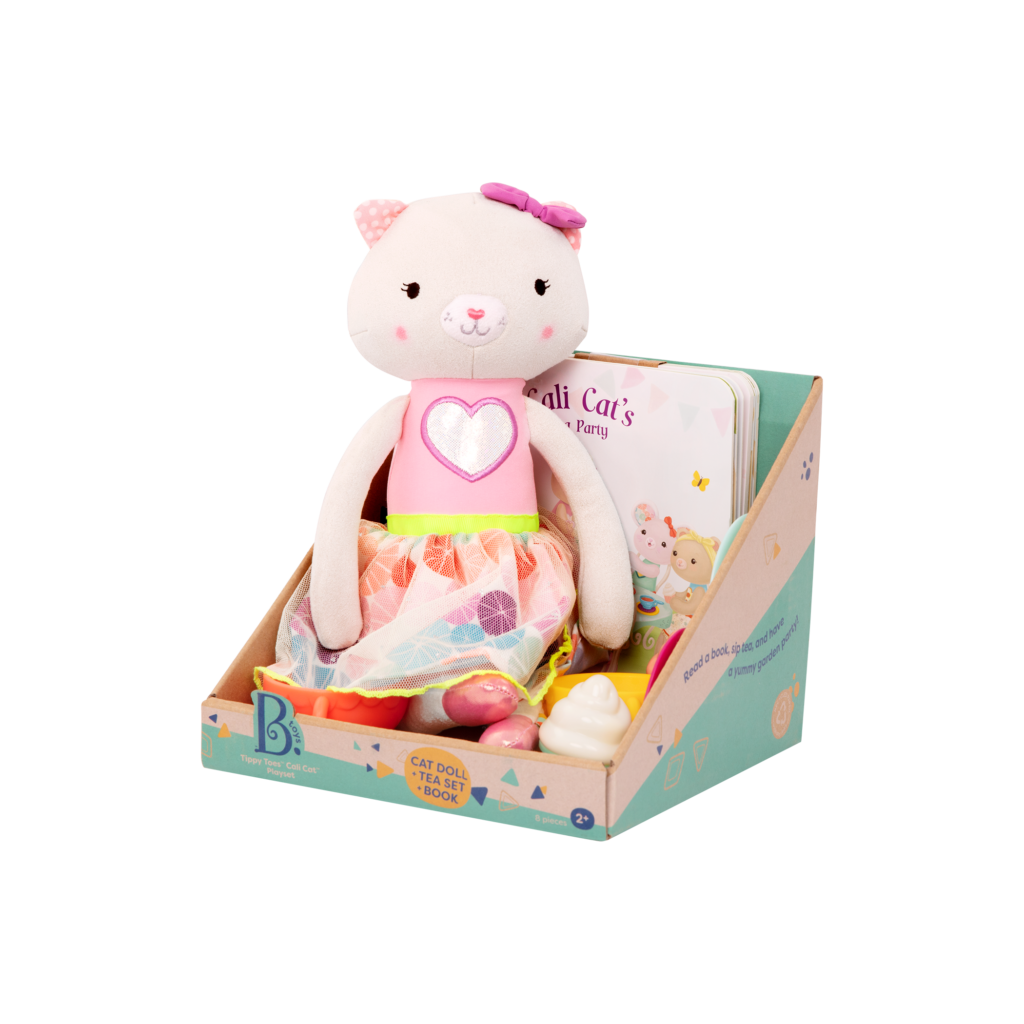This detailed image showcases a child's toy set featuring a plush cat doll nestled inside a turquoise and pink striped container with a distinct sloped back. The front of the box prominently displays the words "cat doll, tea set, and book," with the letter "B" on the bottom left. Adjacent to the "B" is a vibrant yellow-orange circle highlighting the product name. The plush cat doll is primarily pink with distinct features: pink ears, a pink nose, and black eyes with eyelashes. It wears a vibrant outfit including a pink sleeveless top with either a yellow sash or a neon green belt, a heart on the chest, and a colorful skirt with various patterns. The doll’s legs, pink at the tips, extend from beneath its dress. Inside the container alongside the doll are various play items and a booklet titled "Cali Cat's Party" in dark pink letters against a white background. These items include a teacup and saucer, additional bowls, and a small cupcake with white frosting, enhancing the play experience for children.